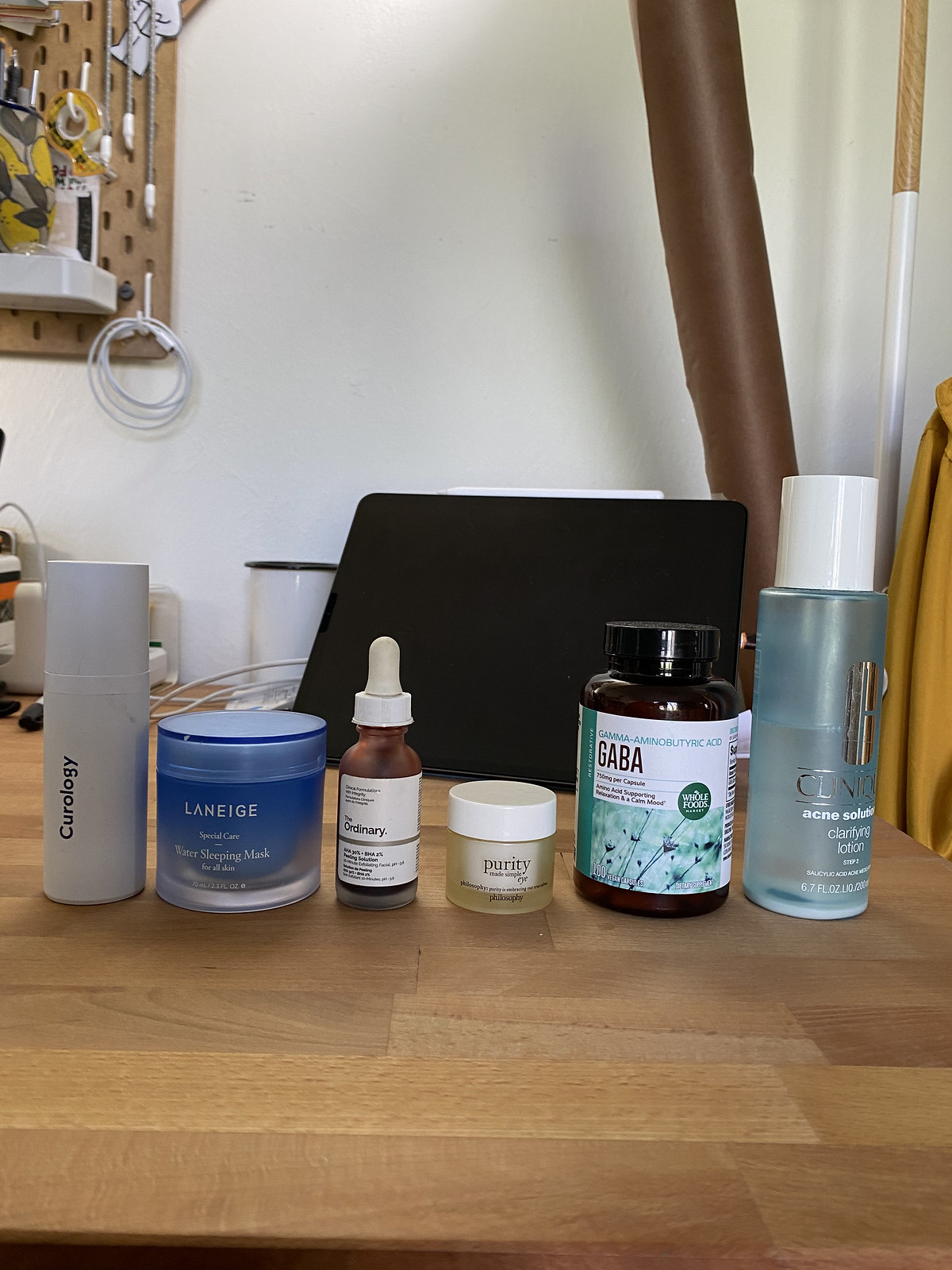In the image, starting from the left, a series of skincare and supplement products are neatly arranged. The third item from the left is the Laneige Water Sleeping Mask, designed for all skin types, known for its hydrating properties. The next product, positioned centrally, is from The Ordinary; however, the specific solution cannot be identified due to the small text on the label. Following this is the Purity Eye treatment by Philosophy, housed in a small canister with a white screw cap, likely aimed at improving the delicate skin around the eyes. Adjacent to it is a bottle of Gamma Amino Butyric Acid (GABA) by Whole Foods, indicating it is a dietary supplement in capsule form. Concluding the lineup on the right is Clinique’s Acne Solutions Clarifying Lotion, a product targeted for acne treatment. Each item is distinctly packaged and clearly displayed for easy identification.